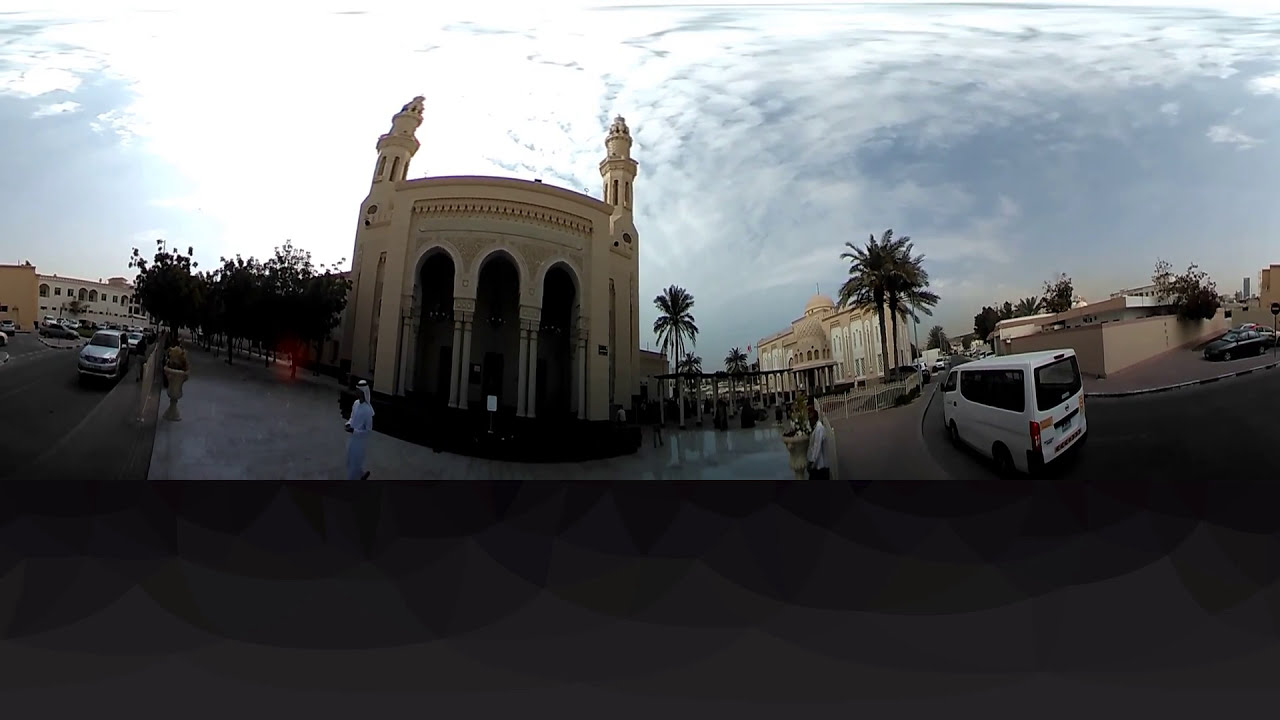This panoramic photograph captures a historic, likely Arabic, building with architectural elegance, including three prominent archways and long empty columns in the middle. The building, made from a beige, sandstone-like material, appears to resemble a temple or mosque, adorned with intricate torches on either side. Surrounding the building, clusters of palm trees are evident, contributing to the exotic feel of the scene. Scattered throughout the photo are several people dressed in traditional clothing, mingling among parked vehicles, including a white van. The sky above transitions from dull blues and grays to patches of white clouds, adding depth to the landscape. To the left and right, smaller buildings emerge from the distance, framing the primary structure and enriching the panoramic view with a blend of cultural and architectural details.